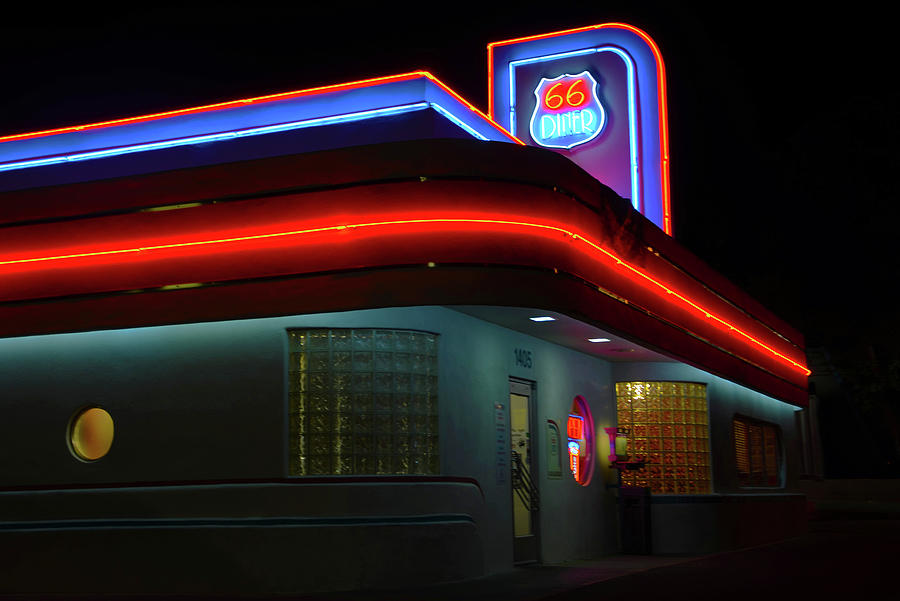This photo captures the nighttime exterior of the 66 Diner, with a striking black background emphasizing its vibrant, nostalgic design. The diner is adorned with red and blue neon strip lights outlining the edges of the roof and building, reminiscent of classic diners. A prominent neon sign atop the building features the iconic Route 66 emblem, with "66" illuminated in yellow within a red circle, and "Diner" in white neon lights. The walls of the diner are a light blue or dark green color, depending on the lighting, and feature distinctive cuboid glass windows that obscure the interior. The entrance door, marked with the number 1405, is also highlighted by neon accents. To the left of the door, a round porthole-like window with a glowing "open" sign adds to the inviting vintage charm.